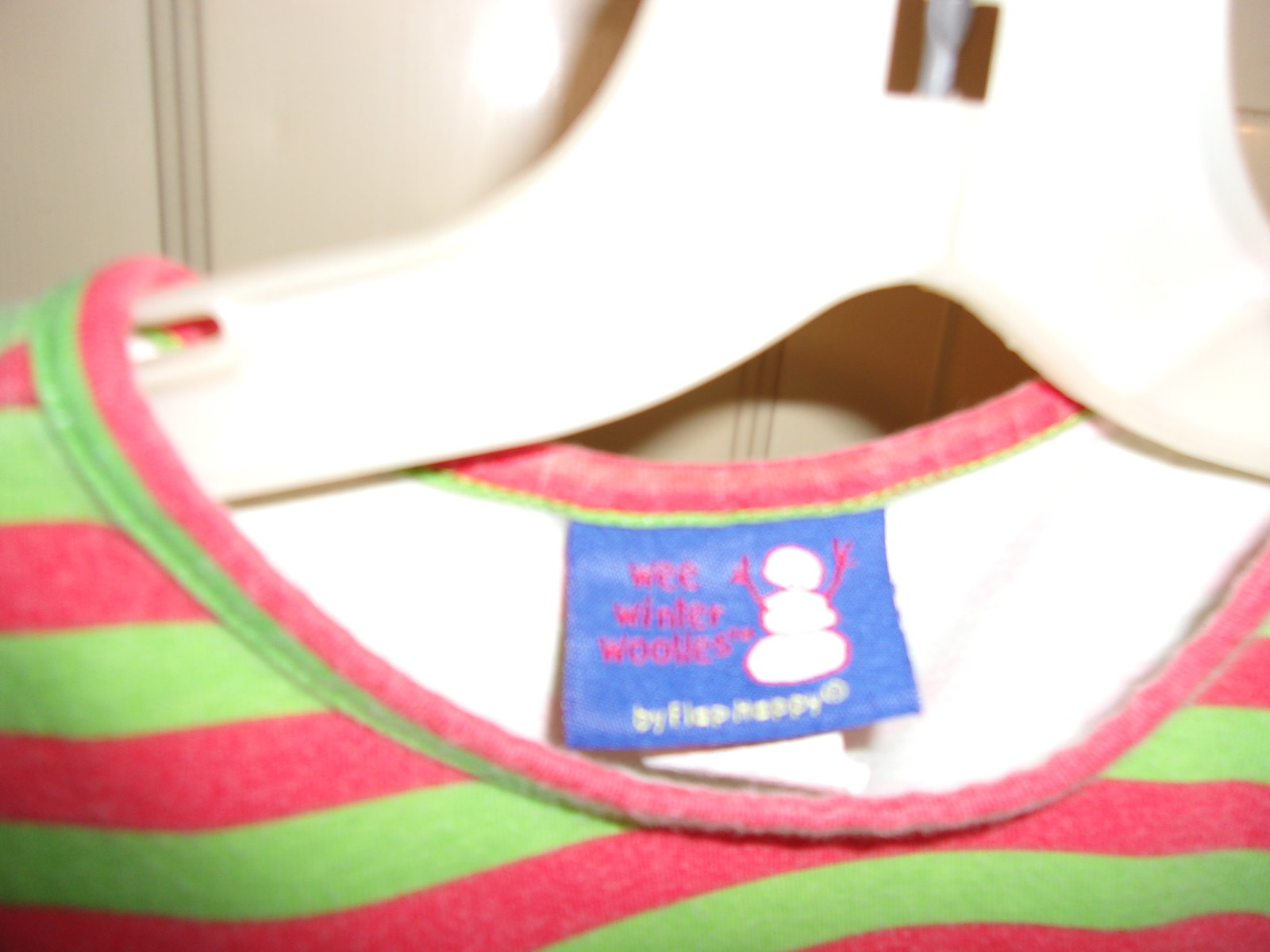The image is a very close-up photograph of a child's shirt on a hanger. Only the collar and tag of the shirt are visible. The hanger, made of thick white plastic, has a unique Y-shape, resembling a boomerang more than the traditional triangle or wire hanger. The shirt itself is striped with alternating light green and candy red colors. The collar follows this pattern, with candy red on the outer portion and green on the inner portion. Behind the shirt is a beige, possibly wooden wall with a slight shine.

The inside of the shirt is white, and it features a blue rectangular tag. This tag showcases a snowman graphic assembled from three white parts, outlined in red with red twig-like arms. Above the snowman, red text is partially legible, appearing to read, "We Winter Wooliness." Below this, in white text, the words "by Flap Happy" are barely discernible. The material of the shirt seems to be cotton or a fuzzy fabric.